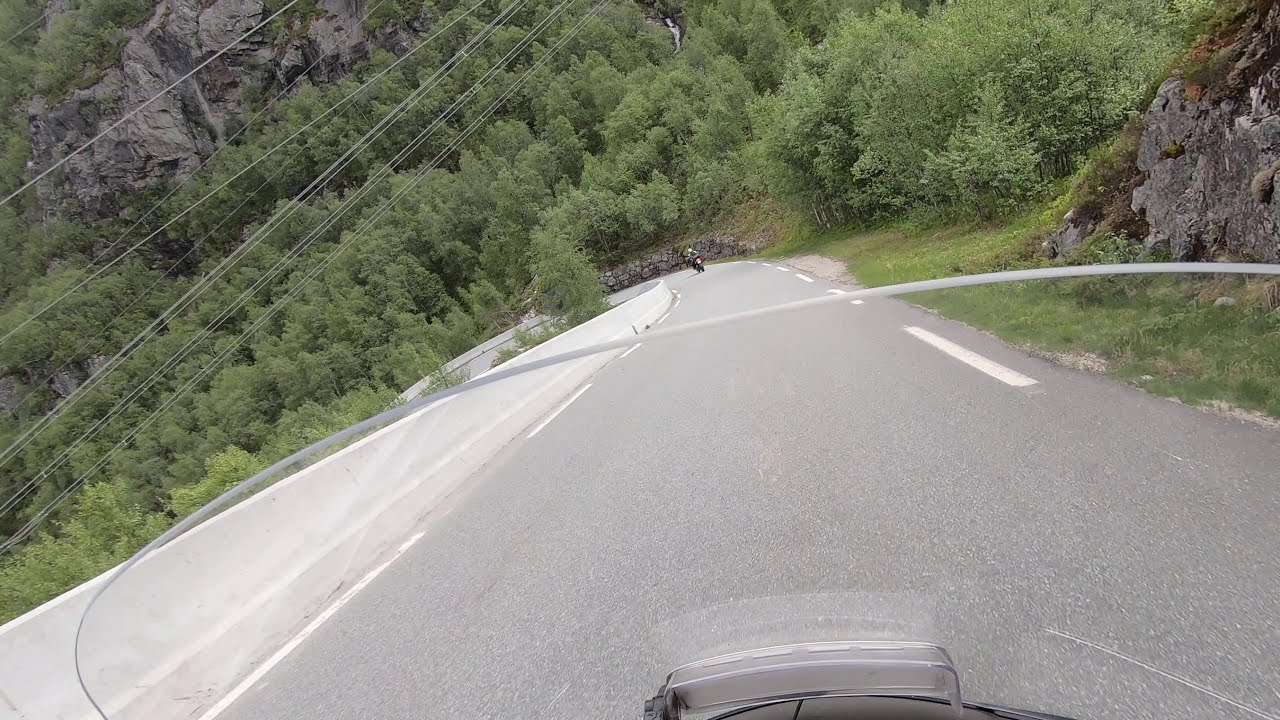This photograph, taken from behind a clear windshield of a motorcycle, captures a scenic view of a forested road. The motorcycle, likely descending a steep, curving hill to the left, is traveling on a single-lane divided highway with a cement guide rail in the center. The road surface is gray asphalt, featuring white stripes, and leads the eye towards another motorcyclist riding ahead in the upper middle of the image. On the right side of the road, there are dense green trees, brush, and a rocky outcropping rising into a mountain. Power lines stretch across the road from the left to the top, adding to the natural and constructed elements in the scene. The image is vibrant with lush greenery contrasting against the gray pavement, depicting a tranquil but dynamic moment of the journey through a picturesque forest.